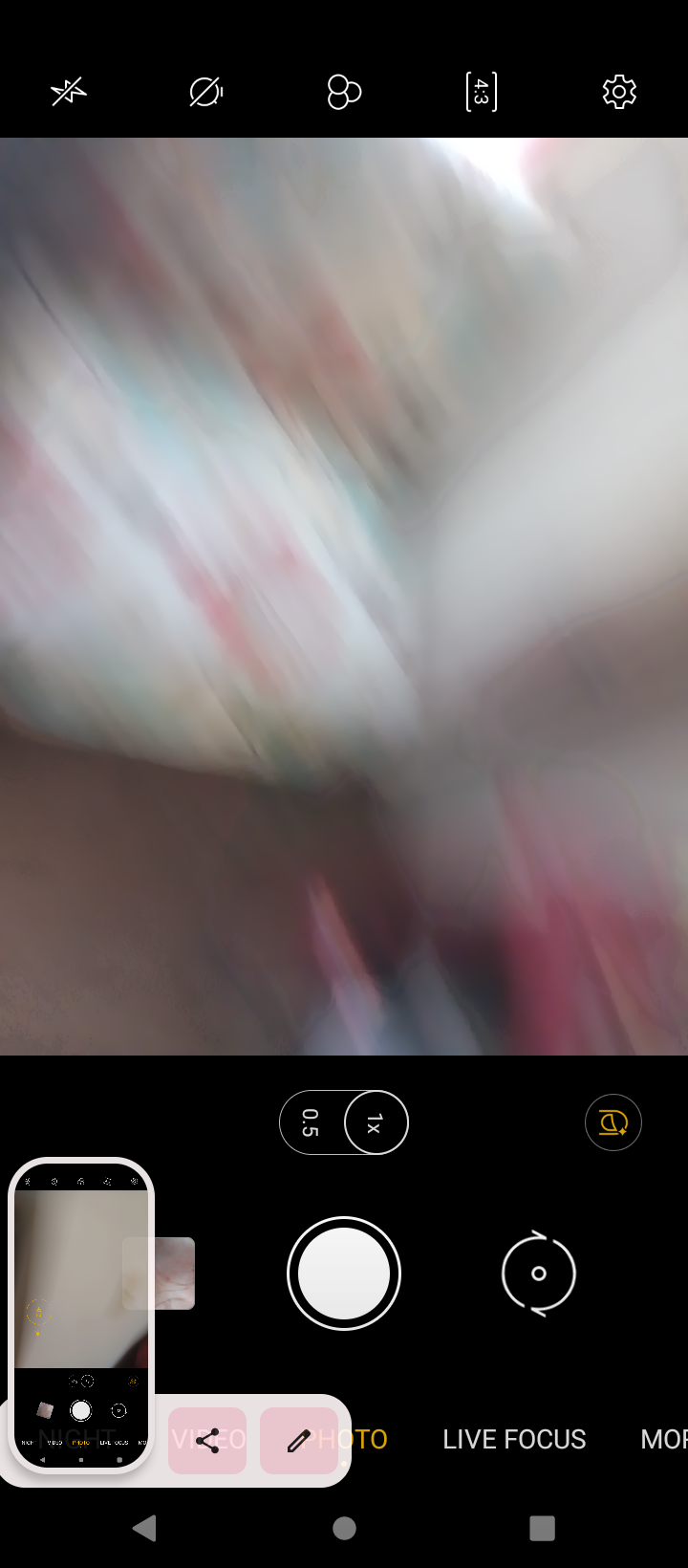On the left side of the screen, there is an image that appears to be a still from a camera interface as it captures a photo. The photo itself is quite blurry, making it difficult to discern specific details. However, it seems to depict a piece of furniture, possibly a chair or a couch, against a wall. The floor beneath the furniture is brownish in color, and there are a few red objects situated in the lower right-hand corner of the screen.

At the top of the camera interface, it is evident that the flash is turned off. Several camera setting buttons are visible, along with a settings gear icon located on the far right. 

Near the bottom of the screen, there is a toggle switch displaying 0.5x and 1x, indicating zoom options. Below this toggle, a camera shutter button is prominently featured, with a dial to its right. The dial is marked in white on a black background. 

Along the very bottom of the interface, there are various mode options like "Photo," "Live Focus," and "Video." Additionally, there is a picture-in-picture display showing a different camera screen in the lower left corner.